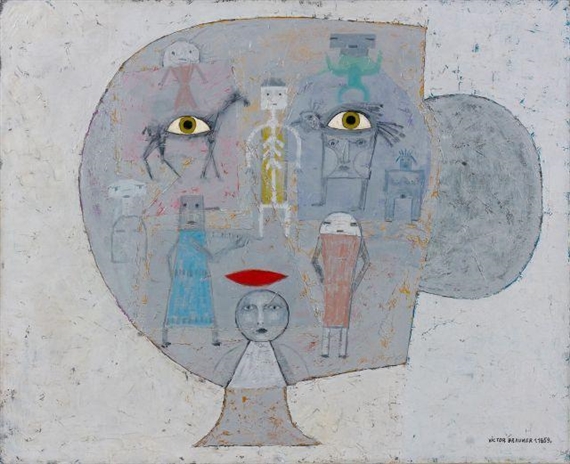This artwork is an esoteric, modern piece that juxtaposes the likeness of a face with multiple smaller faces and figures. The central, irregularly shaped outline of a face is reminiscent of a puzzle piece, incorporating green eyes and red lips. Within this larger face, numerous sketched outlines of people, appearing almost alien or childlike, are interwoven. These sketches feature simplistic circular heads and triangular bodies with stick-like limbs, wearing blue or orange dresses. Among the figures, a smudged outline of a horse is discernible. The overall color scheme of the piece predominantly consists of gray and dark gray tones, accentuated by random blue marks. The bottom right corner bears an illegible signature of the artist, with the possible first name "Victor" and a date, potentially from the late 1950s or early 1960s.